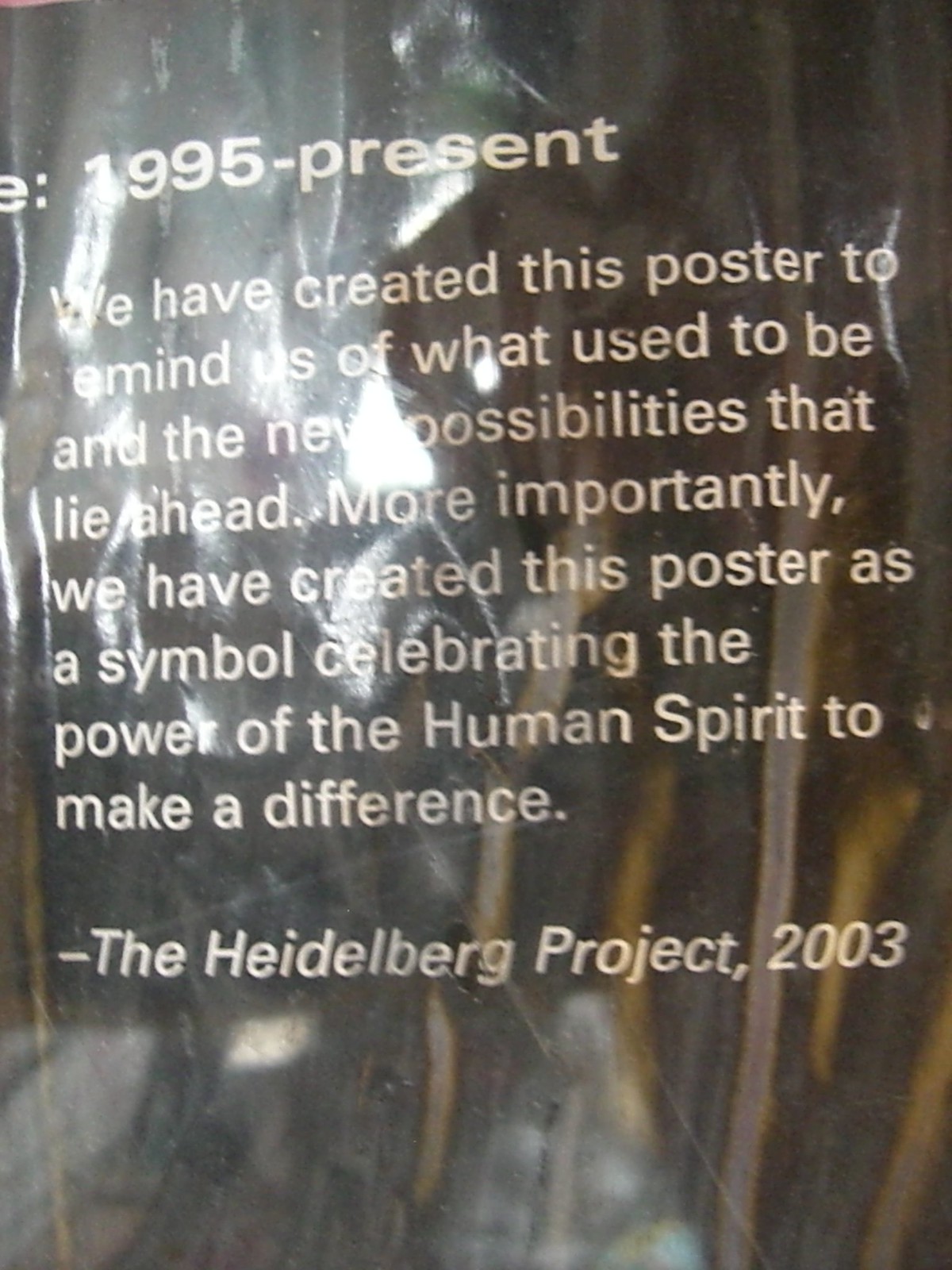The image showcases a close-up view of a poster with a crinkled, reflective surface, characterized by a dark, blackish-brown color. The crinkled texture, scratches, and slight grime obscure reflections, making them indistinguishable, though a light source behind the camera hints at its reflective nature. The white text on the poster reads: "1995 to present", followed by, "We have created this poster to remind us of what used to be and the new possibilities that lie ahead. More importantly, we have created this poster as a symbol celebrating the power of the human spirit to make a difference." Below this, a dash precedes the italicized words, "The Heidelberg Project, 2003," in a sans-serif font. This close-up, distorted view emphasizes the poster's state without revealing further context about its environment or location.